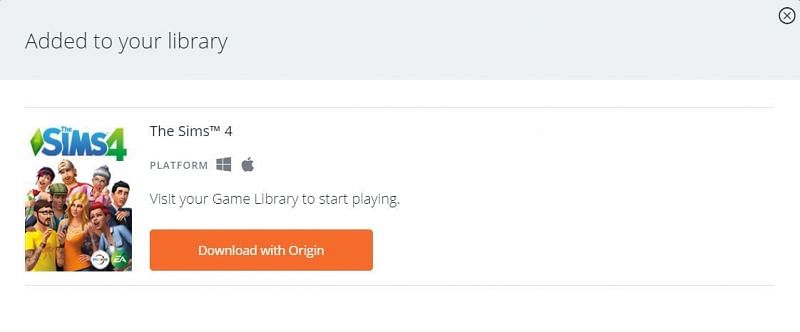This image is a screenshot from the Origin application, closely cropped to highlight key elements. The header is a subtle gray with matching text that reads "Add to Library." In the far right corner, there's a circular button outlined in dark gray with an 'X' in the center, likely functioning as a simple notification close button. Beneath the header, on a white background, is the cover art for the game "The Sims 4." The cover features a diverse group of 3D-rendered humanoid characters of varying ages, ethnicities, and genders, all crowded together. The Sims 4 logo, in blue and green, is adorned with the iconic green plumb bob on its left side. Text below the logo specifies the game as compatible with Windows and Mac platforms, and instructs users to visit their game library to start playing. There is an orange button with white text that says "Download with Origin." At the bottom of the cover, there are logos for Maxis and EA, with the Maxis logo being somewhat unclear due to its small size and white color.